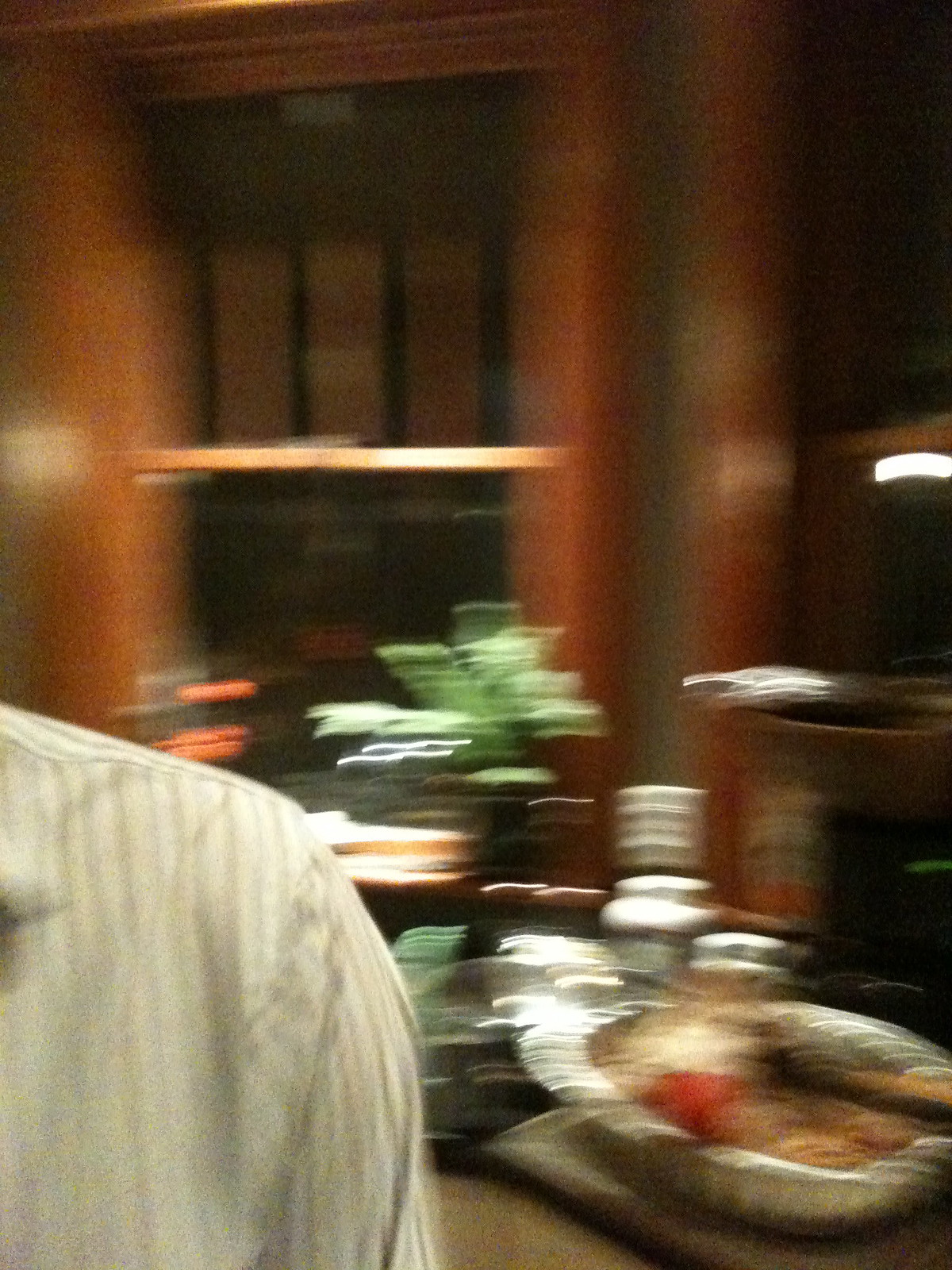The image appears slightly out of focus and is set indoors, characterized by brown paneling on the walls. A tall doorway is visible, and there are black window panes, possibly with coverings, at the top of the image. The lower left corner features the shoulder of a person wearing a white shirt with faint vertical gray stripes. To the right, there's a brown table with a white tray and bowl on it. Inside the bowl, there are items of varying colors—red and brown—with a black spoon resting on top. In the background, a brown counter with white cabinets underneath hosts a silver oval-foil pan containing red, beige, and possibly green elements. Additionally, a green plant in a brown pot sits atop the counter. The scene may suggest a domestic setting with a hint of culinary activity, possibly involving a buffet. Plates are stacked in the corner, and various kitchen utensils are scattered on the table.